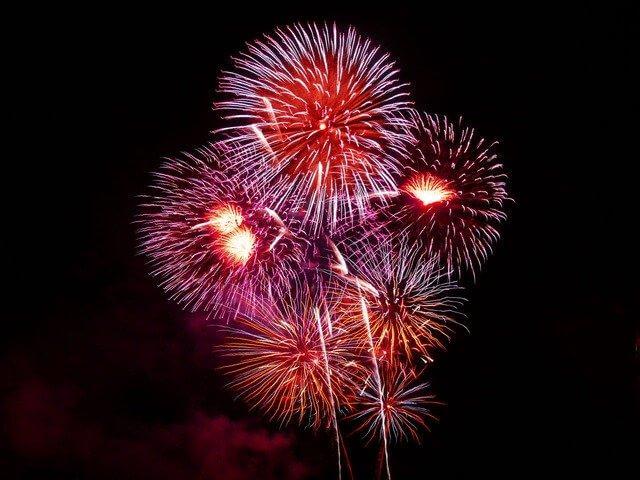In this vibrant, full-color photograph taken outdoors at night, fireworks light up the sky with a spectacular display. The image, distinctly square with no border, is set against the sheer blackness of night, interrupted only by a subtle glow of colored clouds in the lower left-hand corner. At the center bottom, vertical lines reveal the launch of several rockets. From these rockets, six fireworks bursts radiate outward, each displaying a vivid palette of red, white, blue, silver, hints of purple, alongside shades of orange, pink, and yellow. The bursts form intricate, almost floral patterns in the sky, with bright yellow and white streaks adding to the grand spectacle. The smoky residue of the explosions carries tints of red and pink, enhancing the dynamic, colorful experience of this nighttime celebration.